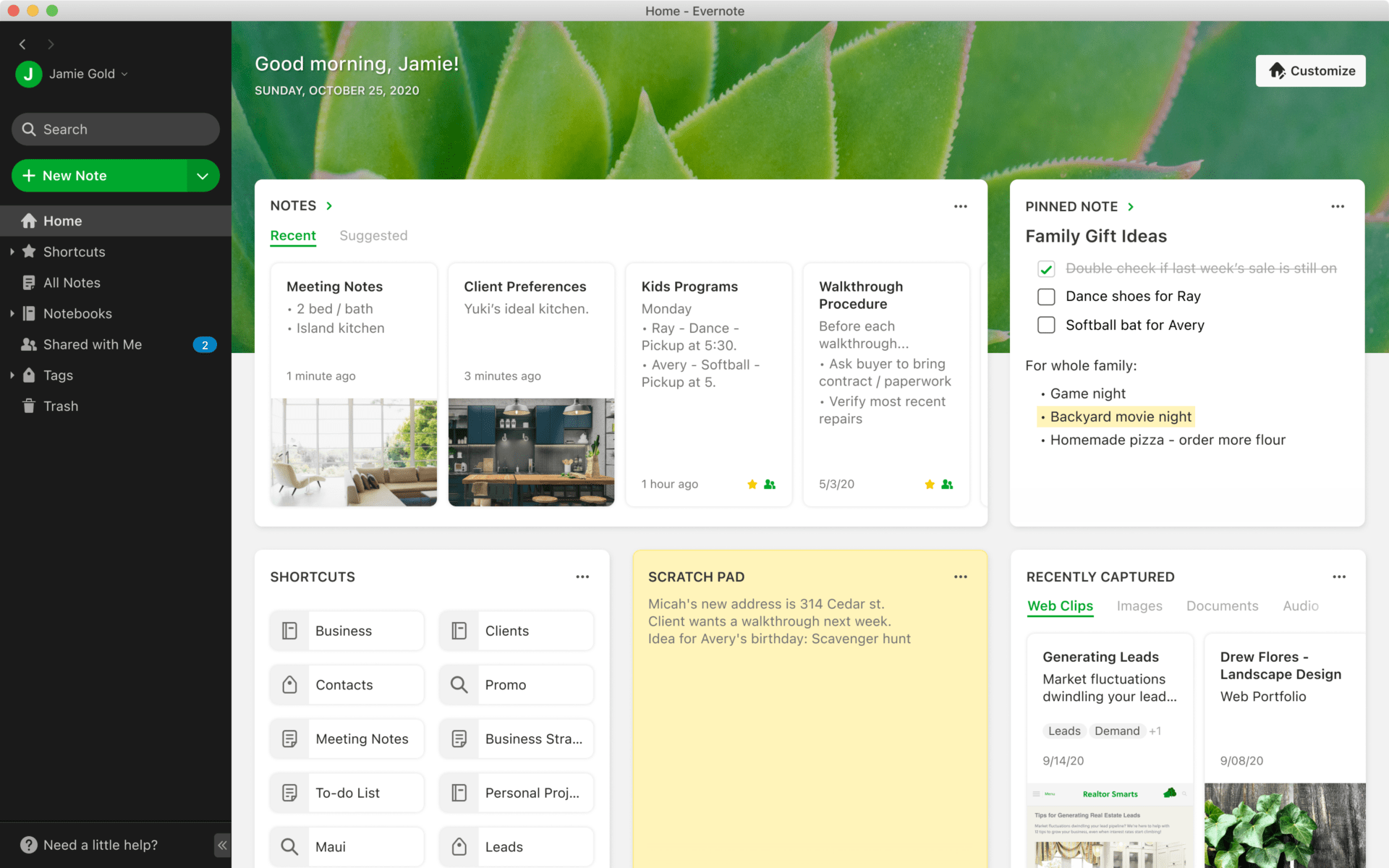The photo is a screenshot from an Apple computer displayed in landscape orientation. At the top of the screen, there is a thin, gray horizontal bar featuring the iconic red, yellow, and green circles in the left corner. Centrally positioned in this bar are the words "Home Evernote."

On the left side of the image, there's a vertical column with a black background. Within this column, there is a highlighted character on the left and a dimmed character on the right at the top. Below this, it displays the name "Jamie Golden White" alongside an avatar, which is a green circle featuring a white "J."

Further down the column, there is a long, oval-shaped gray search bubble with white text inside, followed by a green "New Note" bubble with white font and a plus sign alongside a drop-down caret. Under these elements, there are several options listed with corresponding icons and white text: "Home," "Shortcuts," "All Notes," "Notebooks," "Shared with Me," "Tags," and "Trash." The "Shared with Me" option includes a blue bubble with the number "2," most likely indicating notifications.

The top portion of the main screen displays a background image of leaves with white text overlay that reads, "Good Morning Jamie" and "Sunday, October 26, 2020." It appears to be a web page with the heading "Notes," followed by various subcategories that look like clickable items, potentially including stories.